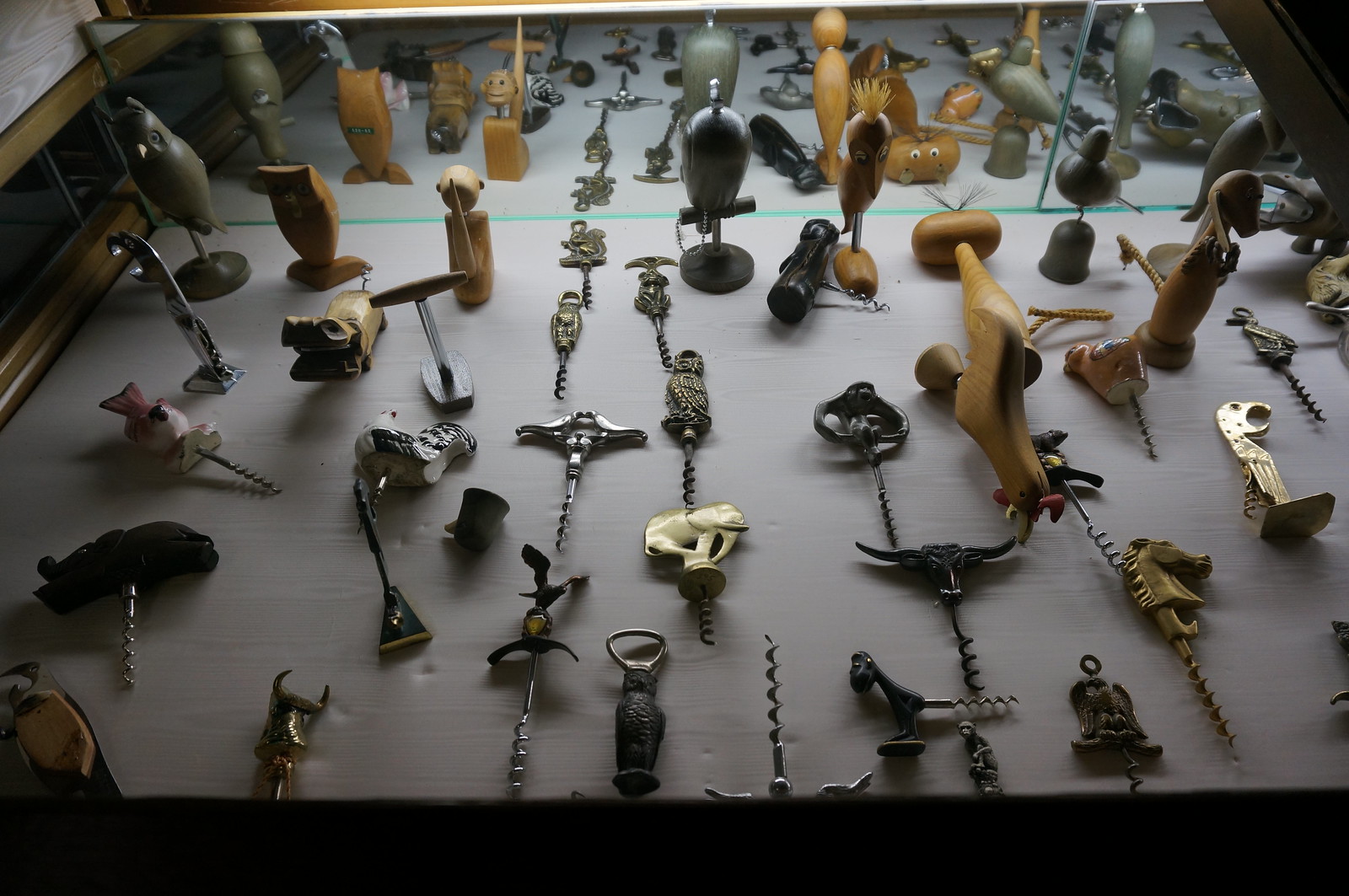This image depicts an elaborate corkscrew collection displayed in a museum. The display case, likely made of glass with a mirrored back, enhances the visual depth of the exhibit, reflecting the intricate details of each piece. The collection showcases various corkscrews of differing sizes, shapes, and colors, with styles ranging from plain metal and wood to detailed animal and character designs. Among the corkscrews are ones shaped like birds, cats, humans, roosters, elephants, bulls, and monkeys, with some adorned with additional decorative elements such as googly eyes. The displayed items include both upright and horizontally laid corkscrews, some featuring light wooden handles, while others sport colorful or gold-bronze finishes. The base of the case appears to be upholstered, showing dents likely made by the corkscrews. This diverse assembly suggests a thematic emphasis on animal and character designs within the corkscrew collection.